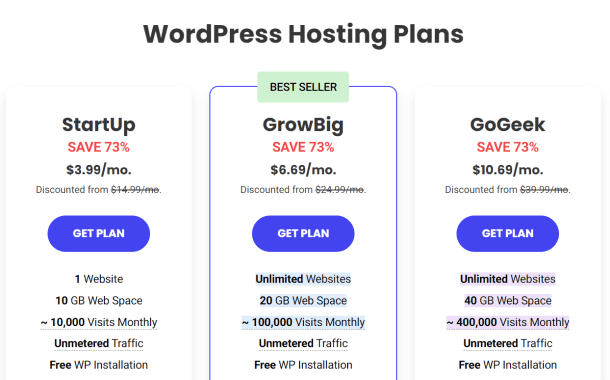The image displays the details of three WordPress hosting plans titled Startup, Grow Big, and Go Geek, arranged from the most affordable to the most expensive. Each plan offers a significant discount of 73%. 

- **Startup Plan**: Priced at $3.99 per month, it is designed for a single website and includes 10 GB of web space, accommodating up to 10,000 monthly visits.

- **Grow Big Plan**: Listed as the Best Seller at $6.69 per month, this plan provides 20 GB of web space and supports up to 100,000 monthly visits.

- **Go Geek Plan**: The most comprehensive option, priced at $10.69 per month, offers 40 GB of web space and can handle up to 400,000 monthly visits.

All plans feature unmetered traffic and free WordPress installation. Each plan also has a prominent "Get Plan" button below its respective price. The image highlights the comprehensive nature and competitive pricing of the hosting options available.